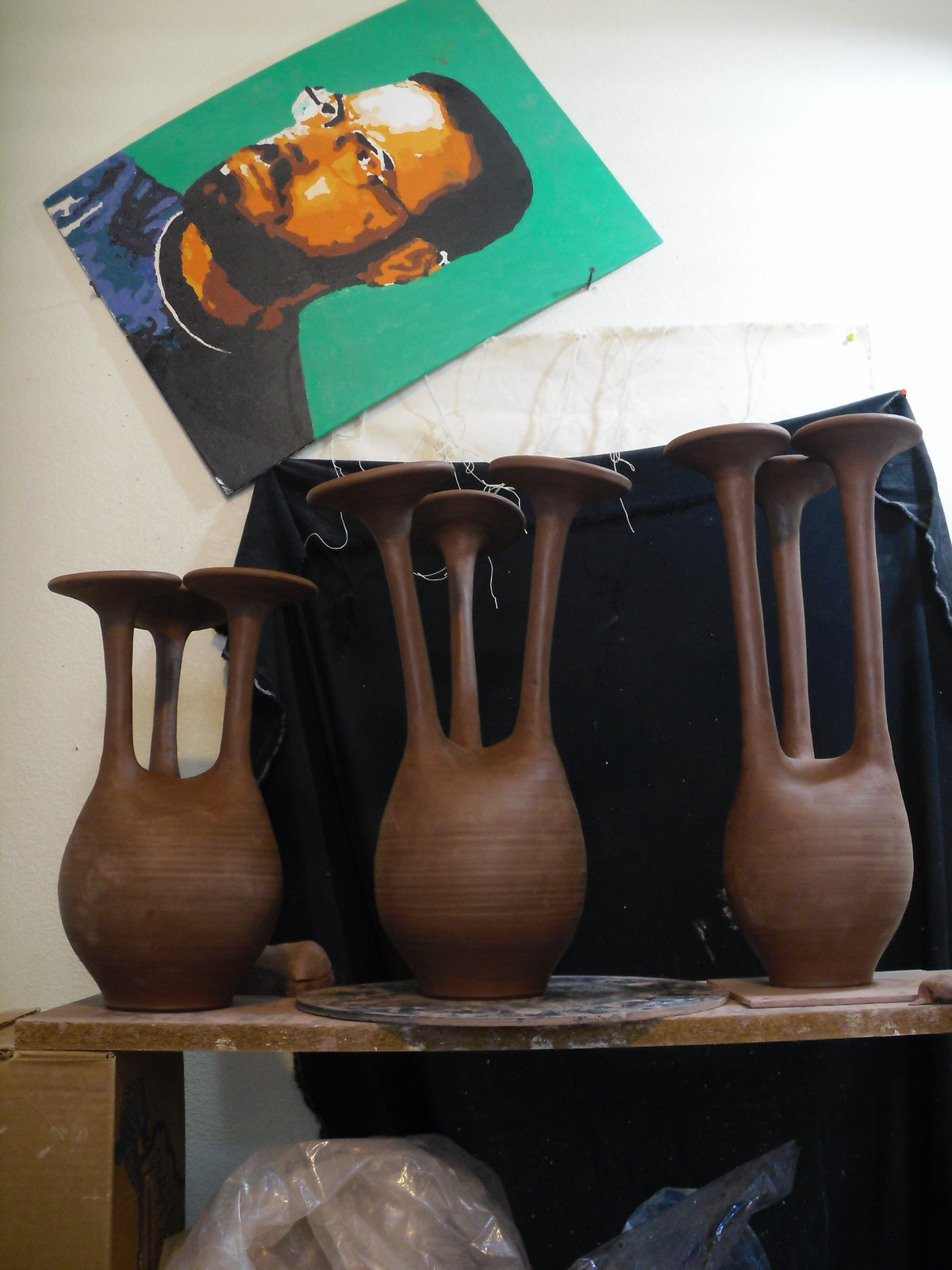The image captures a brown table with thicker legs and a thin top, on which three uniquely designed brown figurines resembling pottery are placed. The bases of these figurines are round, supported by three long, circular poles ending in flat, round surfaces. The figurines vary in size: one is small, another medium-sized, and the third is taller. Behind the table, a black sheet is pinned to the wall with pushpins, partially covering plastic bags that are faintly visible. Above the black sheet, there is a painting featuring a man from the chest up against a green or aquamarine background. The man has short brown hair, a short beard, and glasses, and he is wearing a blue crew-neck shirt with white trim. He appears to be looking to his right. The vibrant color and detailed depiction of the man in the painting provide a stark contrast to the brown and black tones of the figurines and the background.